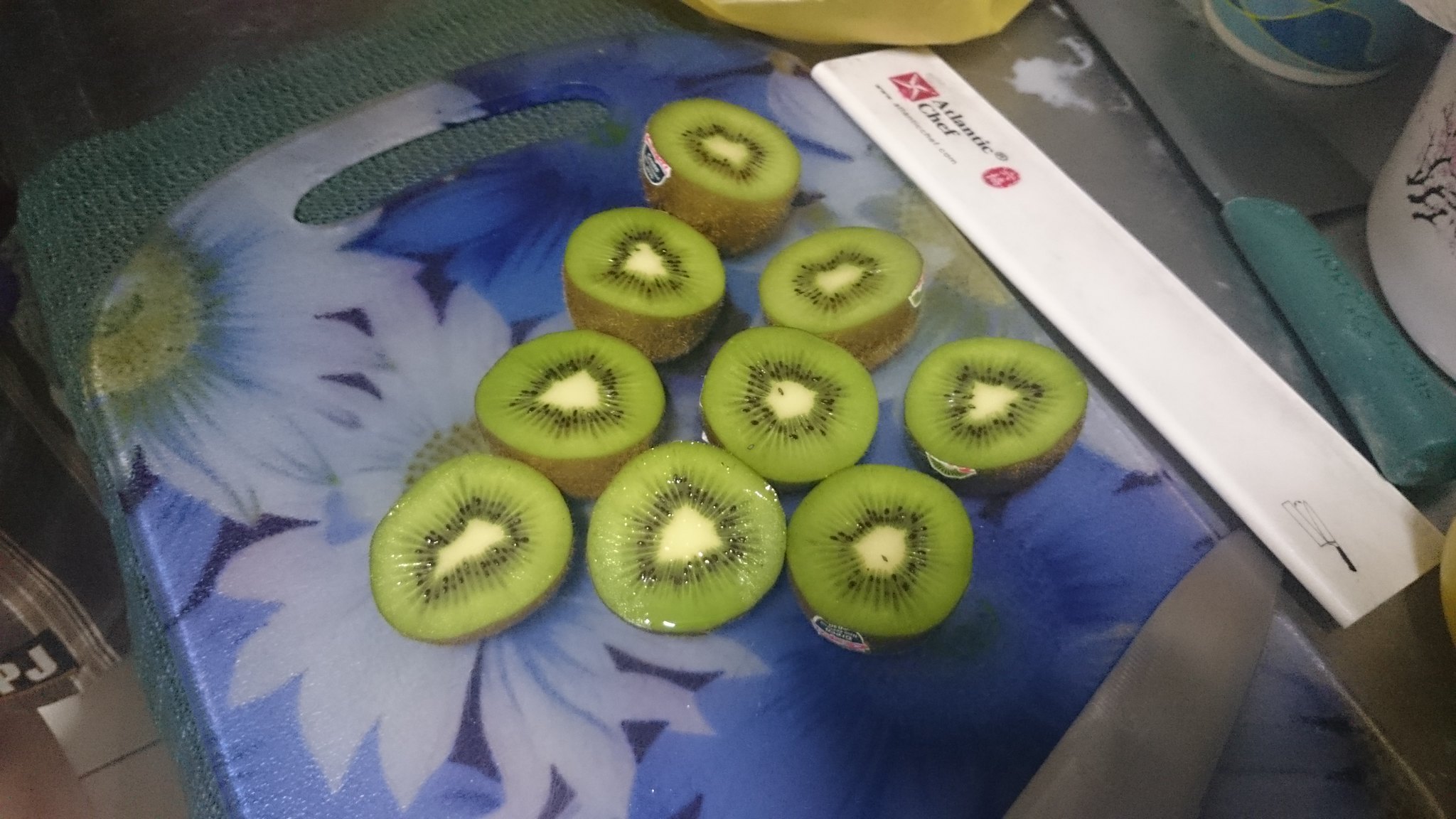The image showcases a blue cutting board with a pattern of large white daisies with yellow centers, positioned at the center of a cluttered kitchen scene. The cutting board is accompanied by a variety of kiwis, sliced into different sizes, forming a triangle pattern that stretches towards the right of the image. The kiwi slices, with their vibrant green flesh, white centers, and surrounding seeds, rest partially on a white sheet of paper or cardboard lying parallel to the cutting board. This paper, which adds to the cluttered ambiance, features red and black text that reads "Atlantic Chef" along with a red logo. The faint shadows cast by other kitchen items add depth to the right side of the cutting board. The handle of the cutting board is visible in the top left-hand corner, indicating its orientation. In the upper right section of the image, partial views of a white coffee mug and another with a blue wavy pattern can be seen. Additionally, a teal-handled butcher knife and another knife blade stretch across the lower right area. The scene suggests a busy kitchen environment, possibly a culinary student's workspace, set against a background of a stainless steel table and a non-slip mat underneath the cutting board.